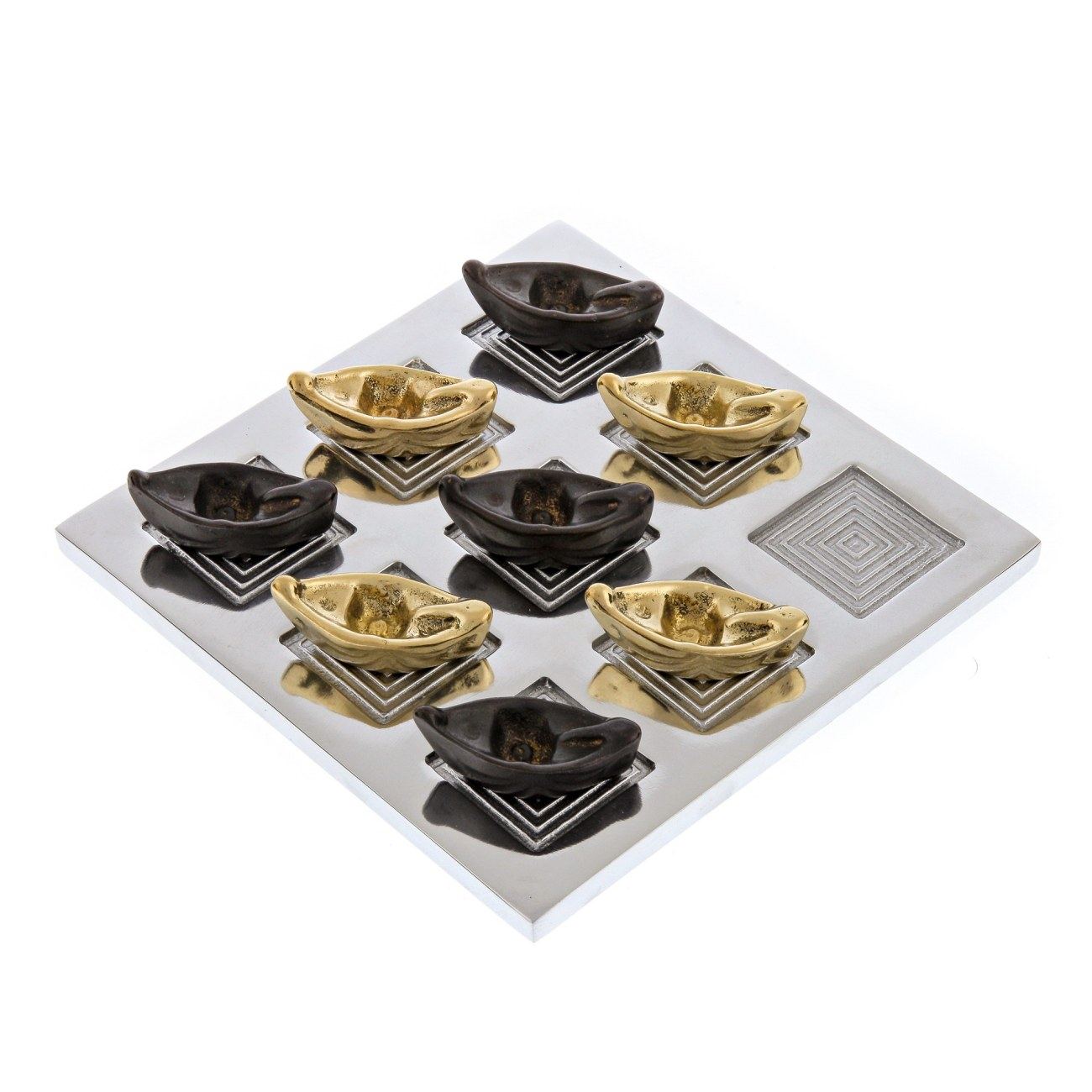The image showcases an artistic display on a silver or stainless steel plate, positioned diagonally like a diamond. The plate features a three-by-three grid of indented squares, each adorned with a geometric border of concentric ridges creating a textured pattern. Placed within these indents are eight boat-shaped objects: four in a rich brown color resembling chocolates, and four in a golden hue that may be chocolates wrapped in vibrant gold foil, sculpted to appear molten and elegant. One square remains empty, adding to the intriguing arrangement. The unique interplay of colors and shapes gives the impression of a luxurious and sophisticated design that could be part of a board game or a decorative piece suitable for a refined setting.